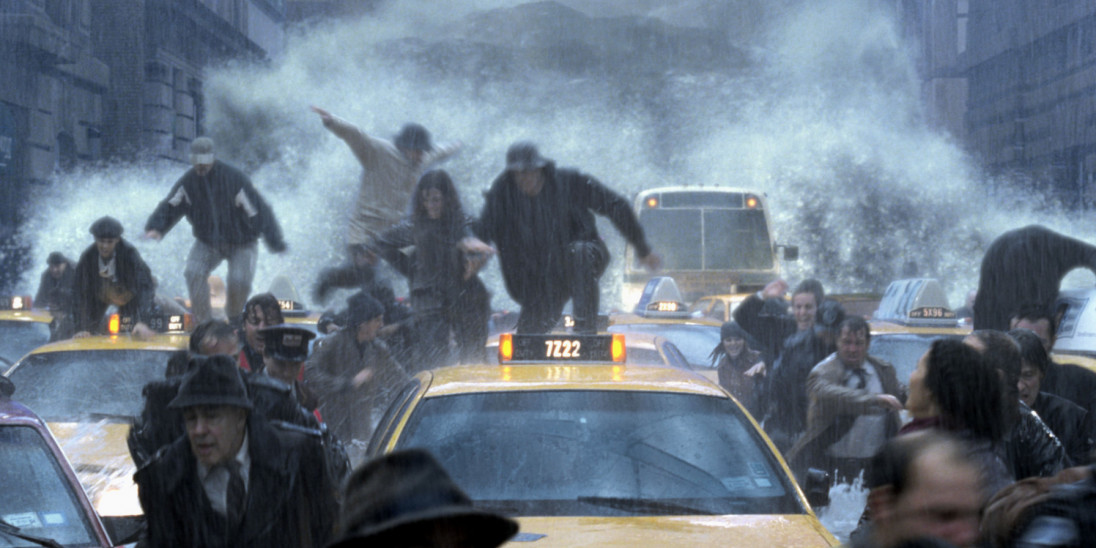This image, which resembles a dramatic still from an action movie, captures a chaotic scene of a bustling city street deluged by a massive flood. The camera faces down a street lined with stone buildings, primarily gray in color, creating a chiaroscuro effect due to the mixed lighting from the wave's reflection. The bright lights on the vehicles and water enhance the stark contrast between illuminated areas and shadowed corners, especially noticeable with the taxis and buses.

Amidst a traffic jam dominated by yellow taxis, many of which feature illuminated numbers like the central taxi marked "7222," and a few cars and a bus in the background, people are desperately fleeing the impending deluge. Most of them, dressed in business attire such as suits, ties, and hats, are abandoning their vehicles and running towards the camera, navigating the cramped spaces between the cars. A few individuals take a more desperate route, clambering over the vehicle roofs in their soaked clothes as water cascades around them. The overall atmosphere is dark and stormy, adding to the sense of urgency and pandemonium as the flood surges through the city, threatening everything in its path.